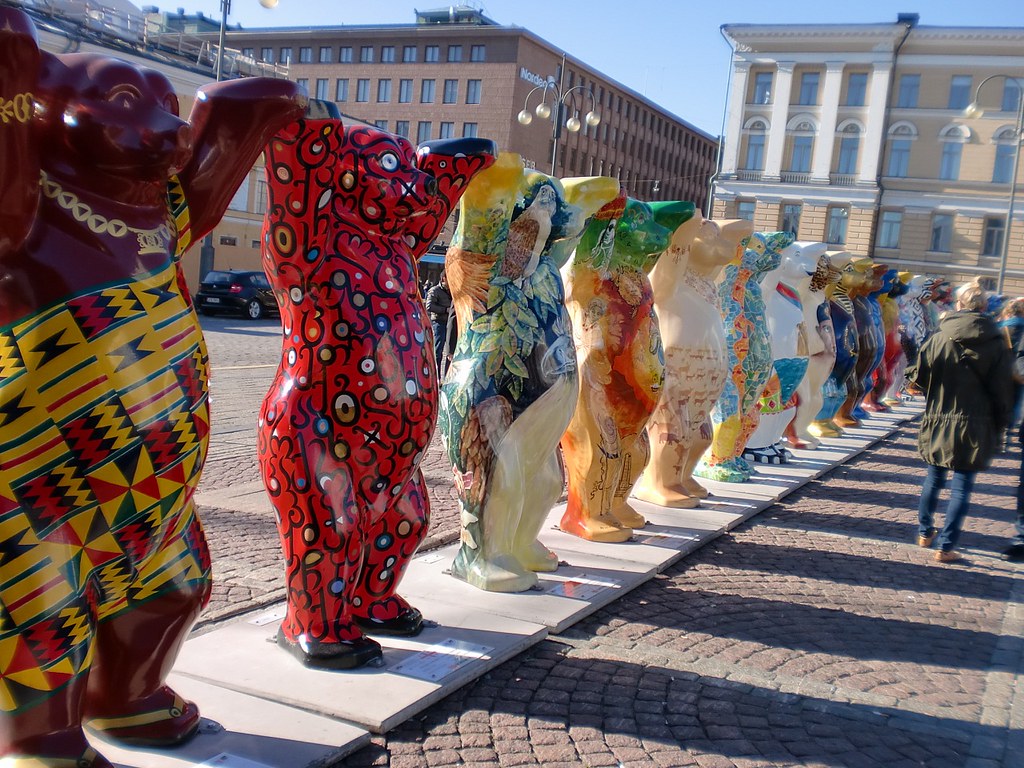This photograph captures an outdoor art display in a city square under a blue sky framed by two large business-like buildings. The main focus is a line of colorful bear statues, each uniquely decorated and standing on square concrete platforms that run diagonally from the bottom left to the upper right of the image. The bears, all molded in the same upright stance with paws raised, measure about six to seven feet tall. They are elaborately painted in a myriad of styles: one brown bear sports a yellow outfit adorned with multicolored designs and a gold necklace, while others feature various themes such as Native American motifs, floral patterns, or ethnic attire. Their shadows are clearly visible on the ground, suggesting a bright yet cool day, as indicated by the few pedestrians dressed in long jackets and pants. The square is paved with bricks and flanked by street lamps and a few parked cars, adding to the urban yet official ambiance of this vibrant public art scene.